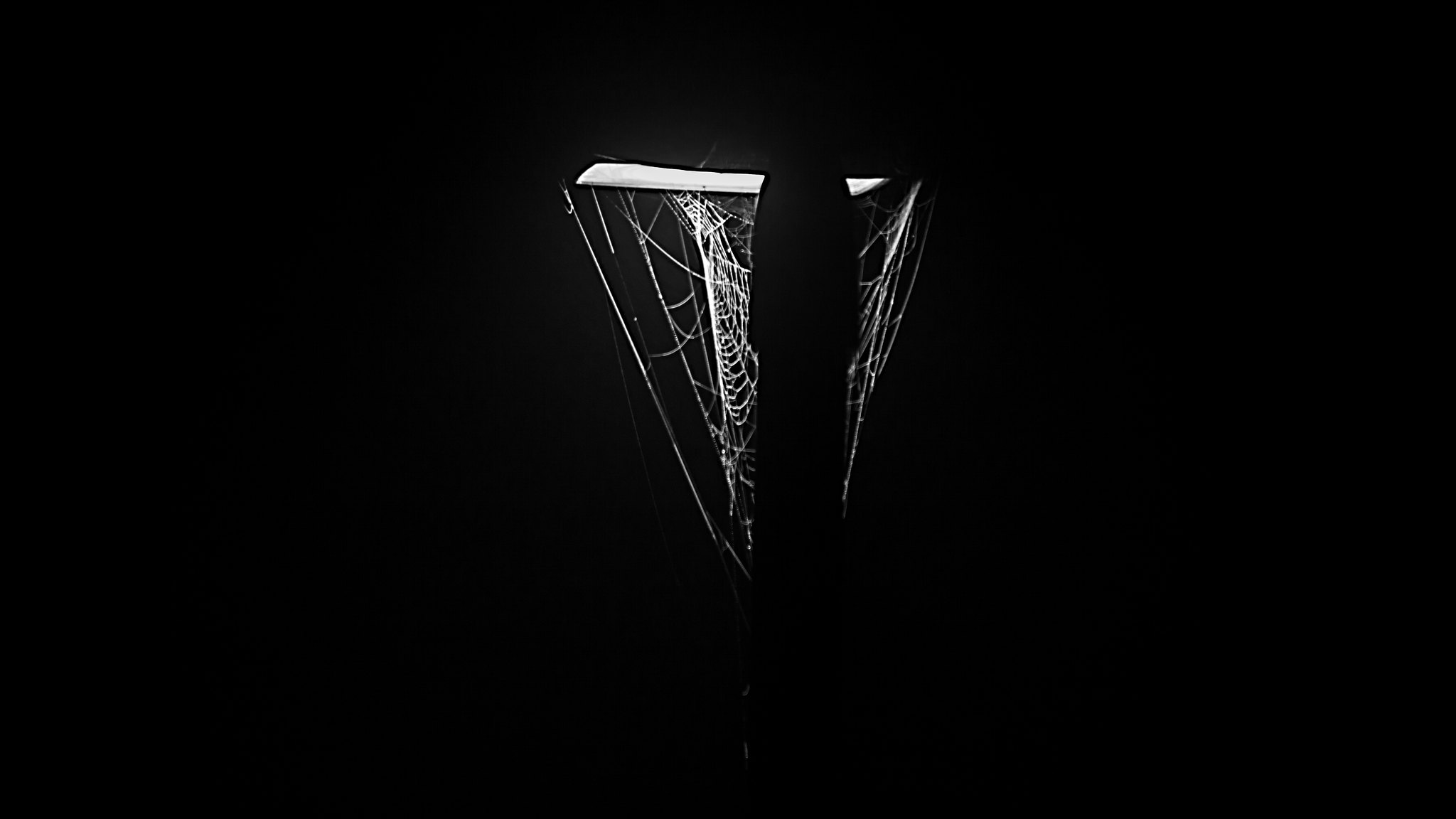The photograph is predominantly pitch black, with a solitary source of light emerging from what appears to be a street light positioned at the top center of the image. Illuminated by this light, a large spider web is visible in the middle of the image, extending both sides and hanging down significantly, suggesting the craftsmanship of an orb-weaver spider. The web is intricately detailed and spans a considerable width, but a tall cylindrical object partially obstructs the light and part of the web, leaving its exact nature indiscernible due to the surrounding darkness. The stark contrast between the brightly lit spider web and the profound darkness creates a hauntingly captivating scene.